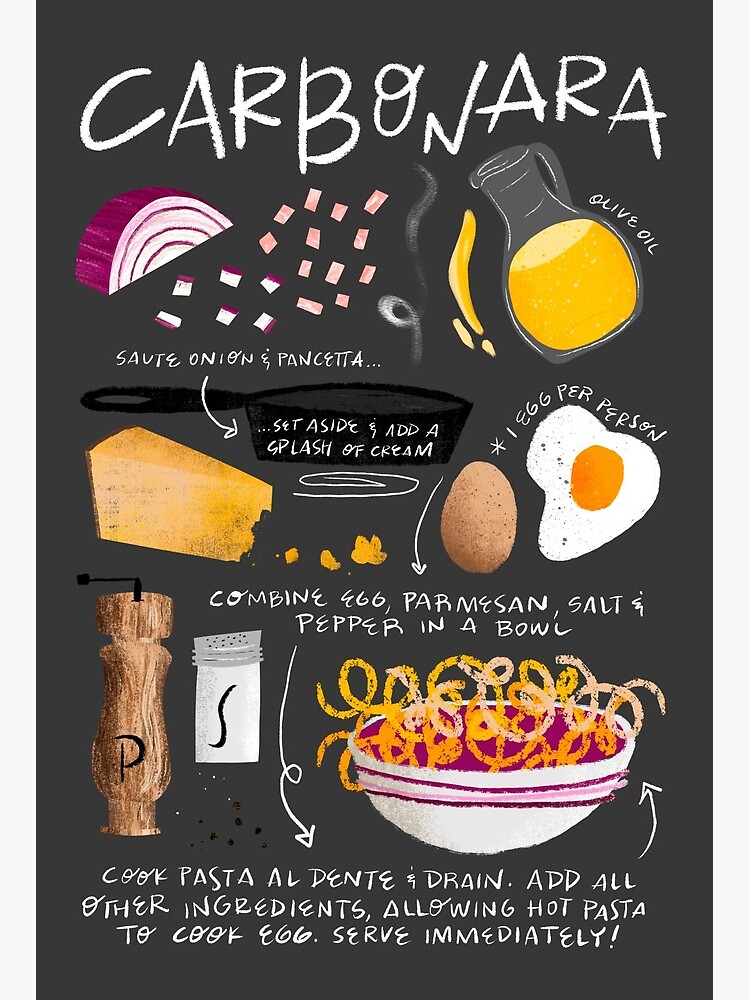The image is a detailed, dark-themed graphic recipe poster for making Carbonara. At the top, the word "carbonara" is written in white against the black background. Below it, a hand-drawn cross-section of a purple onion in a semicircle shape is depicted, alongside small slices of the onion, and the instruction "saute onion and pancetta" is provided. To the right, there's an illustration of olive oil pouring from a tilted bottle, next to a black frying pan with its handle facing left. The instruction next to these images reads, "set aside and add a splash of cream." Below the frying pan, there's a wedge of cheese with a few crumbs beside it, accompanied by a whole brown egg and a cracked egg showing its yolk and white. The instruction here mentions "one egg per person" and directs to "combine egg, Parmesan, salt, and pepper in a bowl." There are also illustrated salt and pepper shakers beside a mixing bowl. At the bottom, the recipe concludes with "cook pasta al dente and drain. Add all other ingredients, allowing hot pasta to cook the egg. Serve immediately."